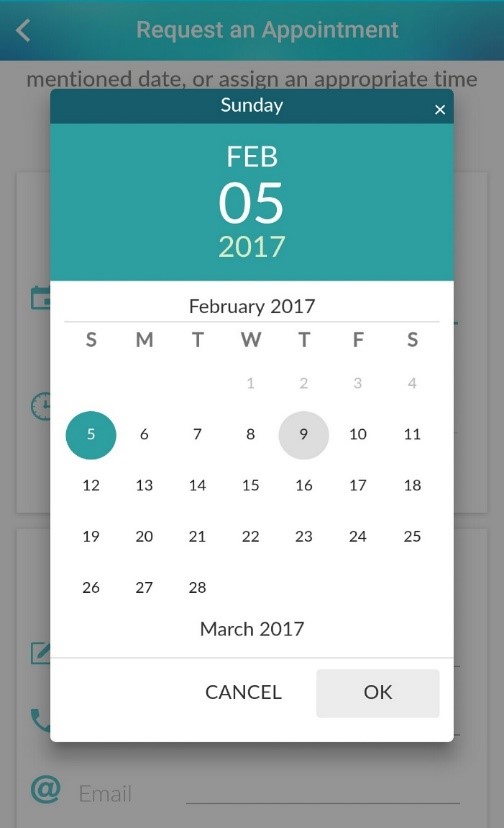The image is a screenshot from a cell phone displaying an appointment scheduling interface. The background has a gray overlay. At the top of the screen is a blue bar featuring a yellow and white arrow pointing to the left. In the center of this bar, the text "Request an Appointment" is written in white.

Below this bar, the interface has a white background overlaid with gray. Black text on this background reads, "mention date or assign an appropriate time." A pop-up window is open in this interface, containing several elements:

- The top section of the pop-up has dark blue text with "Sunday" written in white text at the center. An 'X' icon is situated on the right-hand side to close the pop-up.
- The middle section of the pop-up features lighter blue text. The white text reads: "Feb 05, 2017." 
- This section also contains a calendar with a white background. At the top of the calendar, in gray text, it says "February 2017," followed by the initials of the days of the week: "S M T W T F S," representing Sunday through Saturday.
- The calendar days are displayed starting from Wednesday the 1st, ending on Tuesday the 28th.
- The dates 1st to 4th, representing the previous week, are shown in a very light gray color. 
- The 5th is circled and highlighted.
- Dates 6th to 8th are shown in black, while the 9th is circled in gray.
- Dates 9th to 28th are shown in a darker gray.

At the bottom center of this calendar, the text "March 2017" appears, suggesting a navigation option to the next month. The pop-up also contains two buttons: one labeled "Cancel" in the center and another, slightly grayed out, reading "OK." This completes the detailed description of the image.